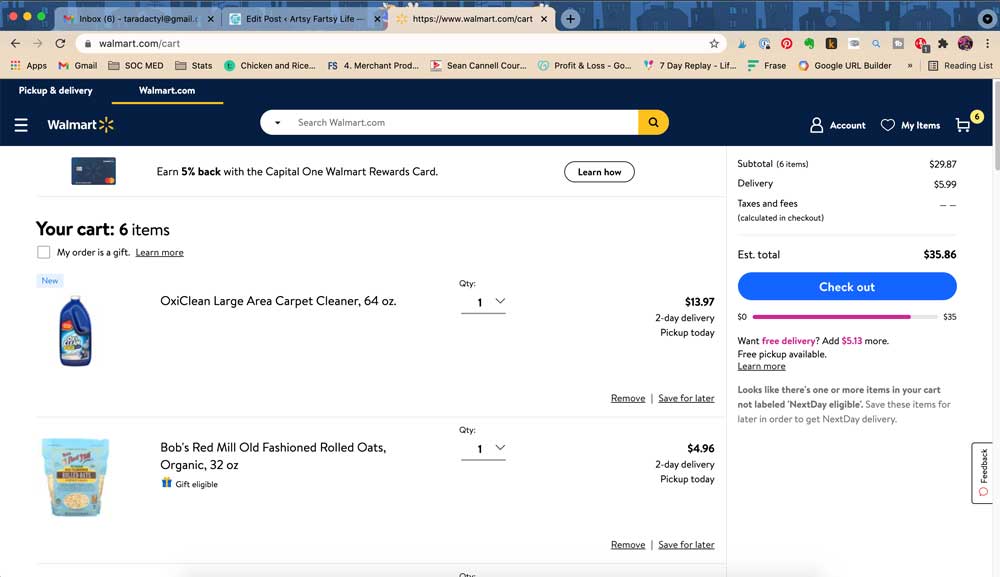Title: Walmart Shopping Cart Page Overview

Caption: The image depicts a shopping cart page from Walmart.com, showcasing a detailed and organized layout typical for online retail platforms. On the left side, the cart indicates a total of six items, while only the top two are visible: one unit of OxyClean Carpet Cleaner and one package of Bob's Red Mill Old-Fashioned Oats. Below the listed items, options for removing or saving items for later are available. 

On the right-hand side, there is a prominent checkout button accompanied by a breakdown of the total cost, including delivery charges and information on the additional amount required to qualify for free delivery or pickup. The page's overall background is white, with the top navigation bar distinguished by Walmart's signature dark blue color. Above the cart, an advertisement promotes the Walmart Rewards Card, highlighting the potential to earn 5% cashback on purchases. The upper menu bar also features several open tabs, enhancing the user navigation experience.